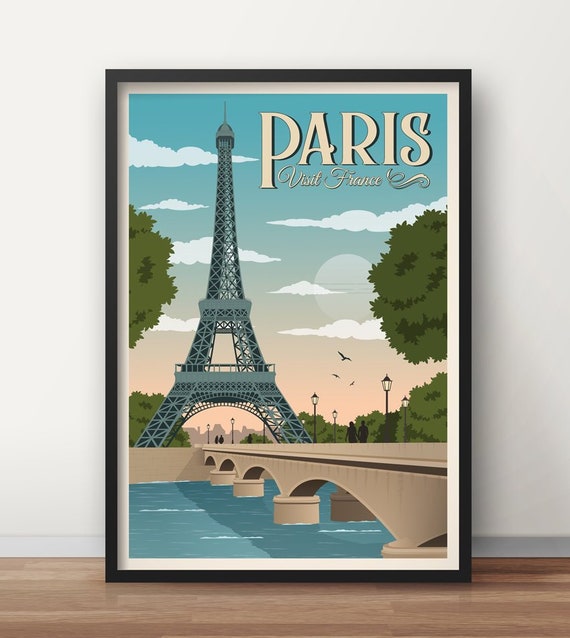On display against a light gray and white-trimmed wall with a wood laminate floor, we see a large framed illustration leaning against the wall. The picture features a simplistic black frame with a white border that enhances the central image, resembling a tourism postcard. The illustration, likely a drawn or rendered creation, showcases the Eiffel Tower prominently centered in a portrait layout. The scene around the Eiffel Tower includes a bridge from the right leading back towards it, spanning a waterway underneath. Silhouettes of people, elegant street lamps, and a variety of trees populate the left and right sides of the image. The sky above transitions from an orange hue near the horizon to a clear blue towards the top, featuring subtle clouds and a faded sun. In the upper right corner of the illustration, bold, stylized capital letters spell out "Paris," with an elegant cursive script below reading "Visit France," although there seems to be a slight confusion in one account mentioning "Visit Florence." The combined elements create a picturesque and inviting depiction of Paris, ideal for a tourism promotion.